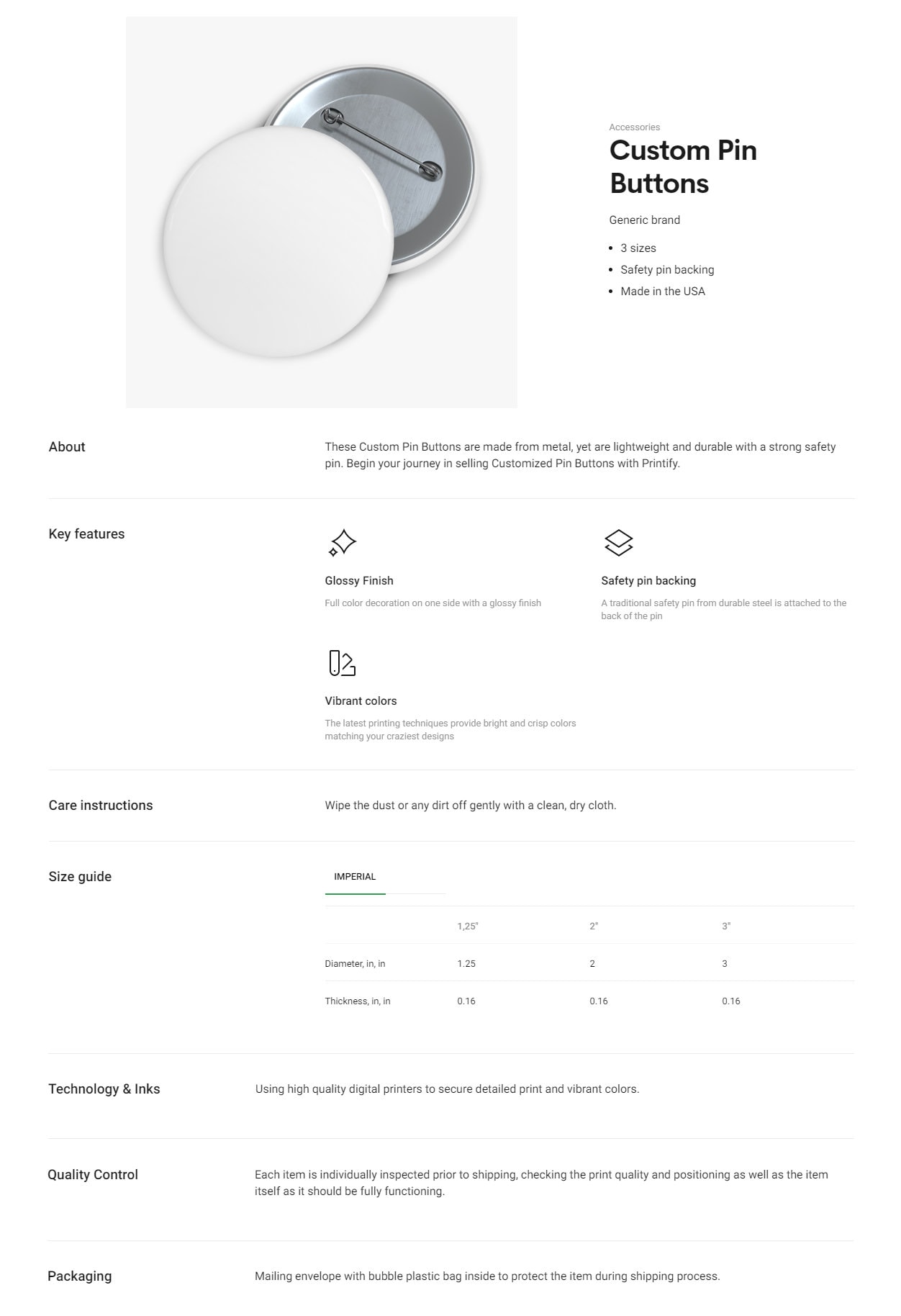The image depicts a webpage dedicated to selling custom pin buttons. At the center of the page is a prominent, large photograph of a circular pin button, designed to be fastened onto shirts and other materials using a pin attached to its back. Users might utilize these buttons for purposes such as campaigns or personalized decorations featuring various images on the front.

On the left side of the image, the text "Custom Pin Buttons" stands out in large font. Beneath this heading, smaller text provides further details, indicating that the pin buttons are from a "Generic Brand," available in "3 sizes," feature "Safety Pin Backing," and are "Made in USA." Further information on the product is organized into vertical sections labeled "About," "Key Features," "Care Instructions," "Size Guide," "Technologies and Links," "Quality Control," and "Packaging." However, the rest of the text on the webpage is too small to decipher clearly, even when attempting to enlarge the image, resulting in some information remaining hidden or distorted. Notably, the webpage lacks any details about the company responsible for selling these custom pin buttons.